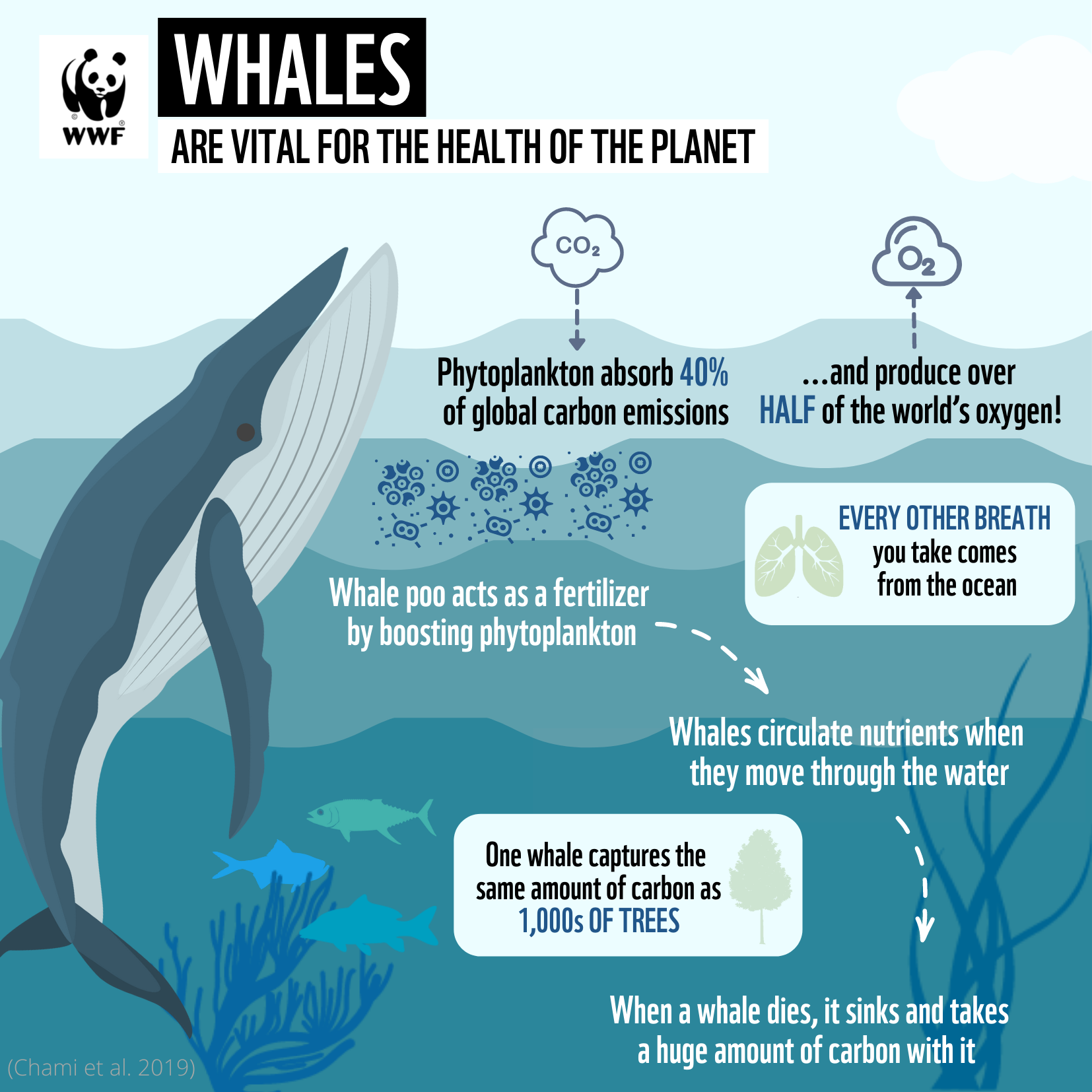This square infographic features a detailed, graphic-style drawing of a gray and white whale peeking out from the ocean surface. The image is set in an aquatic environment with various shades of blue depicting different ocean layers. Vegetation and fish are visible under the water. At the top left corner, there is the WWF logo with a panda bear, followed by the caption in bold text, "Whales are vital for the health of the planet."

The whale is depicted with its head and tapered nose rising from the bottom left to the top middle of the frame. Underneath the whale are three fish and underwater plants. To the right of the whale, a series of informative text bubbles and arrows explain the ecological importance of whales. 

A cloud labeled "CO2" with an arrow pointing down indicates that phytoplankton absorb 40% of global carbon emissions. Below that, a cloud labeled "O2" states that phytoplankton produce over half of the world's oxygen. Another bubble explains that "Every other breath you take comes from the ocean."

Further down, text indicates that "Whale poo acts as a fertilizer by boosting phytoplankton populations." An arrow points to the caption, "Whales circulate nutrients when they move through the water." Finally, a statement at the bottom highlights that "When a whale dies, it sinks and takes a huge amount of carbon with it," and that "One whale captures the same amount of carbon as thousands of trees."